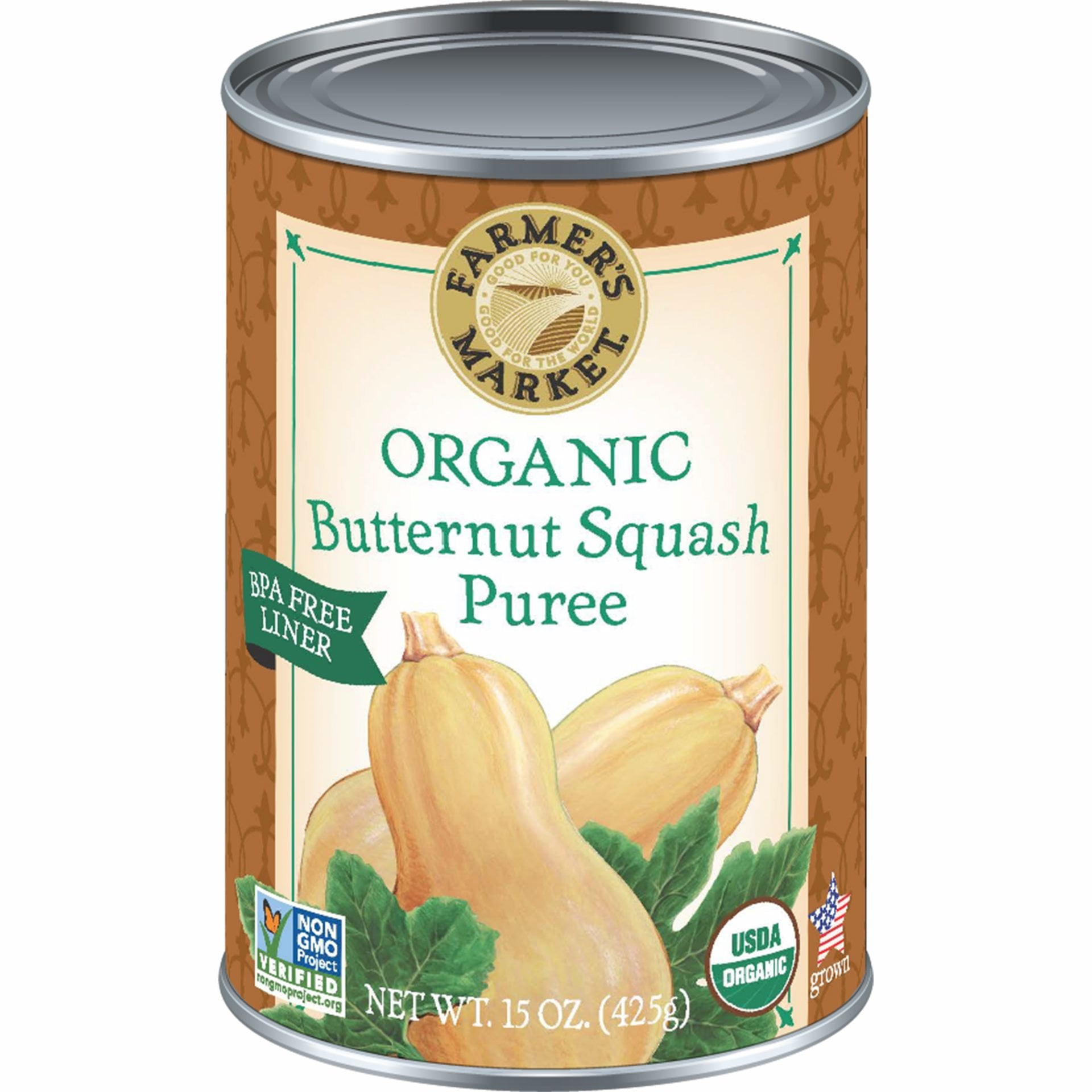This image depicts a can of organic butternut squash puree with a metallic lid typical of canned goods requiring a can opener. The can is primarily brown, adorned with various labels and logos emphasizing its health and environmental benefits. The front of the can features a white rectangular box housing green text that reads "Organic Butternut Squash Puree," accompanied by cartoon illustrations of two tan-colored butternut squashes surrounded by green leaves.

At the top of the can is the "Farmers Market" logo set within a goldish-yellow circle that includes an image resembling sand dunes and a sunrise, alongside the tagline "Good for you, good for the world." 

Additional key information on the can includes:
- A BPA-free liner notice on the left side.
- Non-GMO Project Verified certification and the USDA Organic seal towards the bottom left and right, respectively.
- An American flag within a star icon near the bottom, indicating that the produce is USA-grown.
- The can contains 15 ounces (425 grams).

This detailed labeling is framed by a brown background with various shapes, underscoring the product's organic and American-grown attributes.